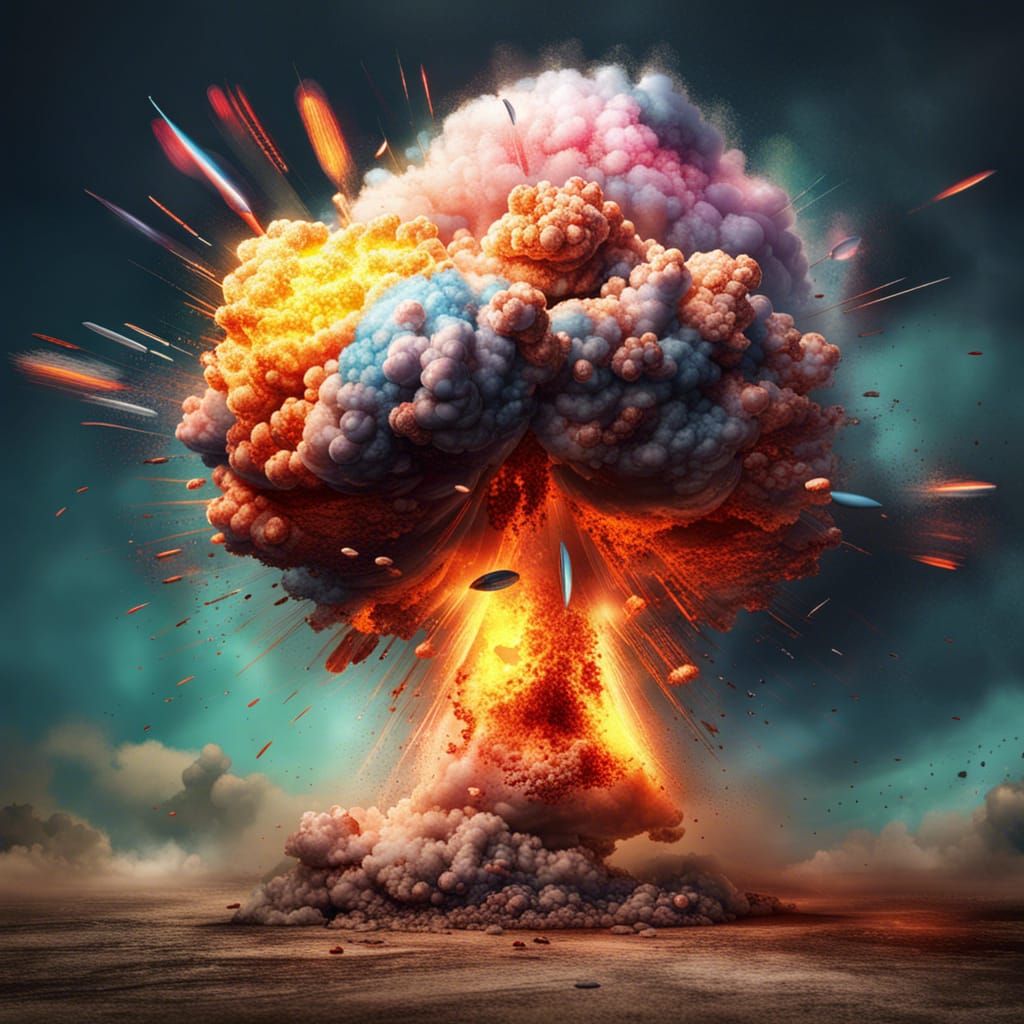The image illustrates a severe and massive explosion, resembling the aftermath of a bomb detonation, possibly nuclear. The base of the artwork depicts brown dirt and plumes of dark brown smoke being forcefully kicked up. Centered in the image is an intense explosion, characterized by bright orange and red hues that give way to a multicolored mushroom cloud. The mushroom cloud's top exhibits vibrant and unusual colors, including blue, yellow, pink, and orange, deviating from typical explosion tones. Rays of light and projectiles emanate from the explosive core, adding dynamic energy to the scene. The background features a bluish, blurred tinge that transitions to a dark or black sky, enhancing the dramatic effect of the digital artwork. The surrounding area near the base appears brown or grayish, while the overall composition highlights the chaotic interplay of various smoke colors and light bursts, underscoring the destructive power of the explosion.